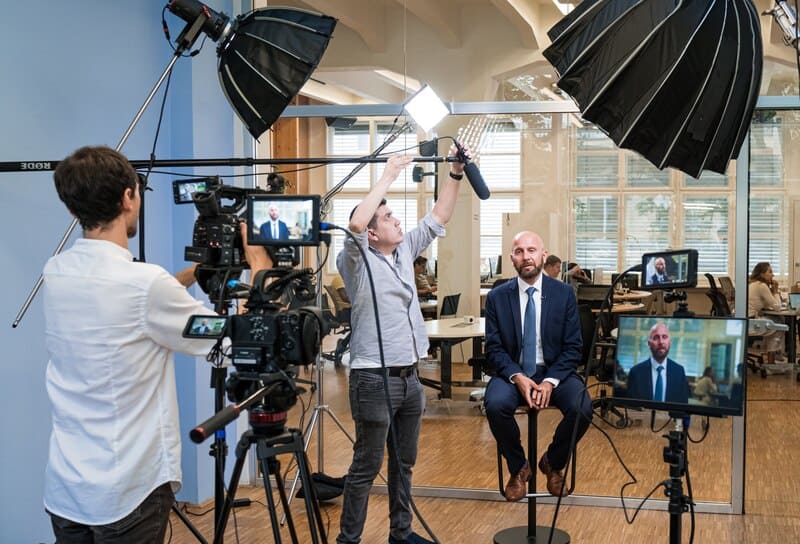In this detailed office scene, a man in a dark blue suit with a matching blue tie and brown shoes is poised on a stool, preparing for a television interview. He has a distinct look with a mustache, a beard, and no hair. Surrounding him are five cameras, each mounted on different stands, capturing his image from various angles. The cameras are black, as are the two umbrella lights that illuminate the area to enhance visibility. There's also a prominent square light overhead, providing additional brightness.

To the right of the man on the stool, a cameraman in a white shirt and dark jeans is meticulously adjusting his equipment. Meanwhile, to the left, another technician in a gray shirt and denim jeans is fine-tuning the microphone setup above the interviewee. Adjacent to the cameraman wearing white, there's a light blue wall, while a transparent glass wall behind the scene offers a glimpse into the office's bustling atmosphere. Through this see-through wall, employees are visible working at white desks, with computers and scattered tables. Windows fitted with blinds further frame the dynamic background of the office space.